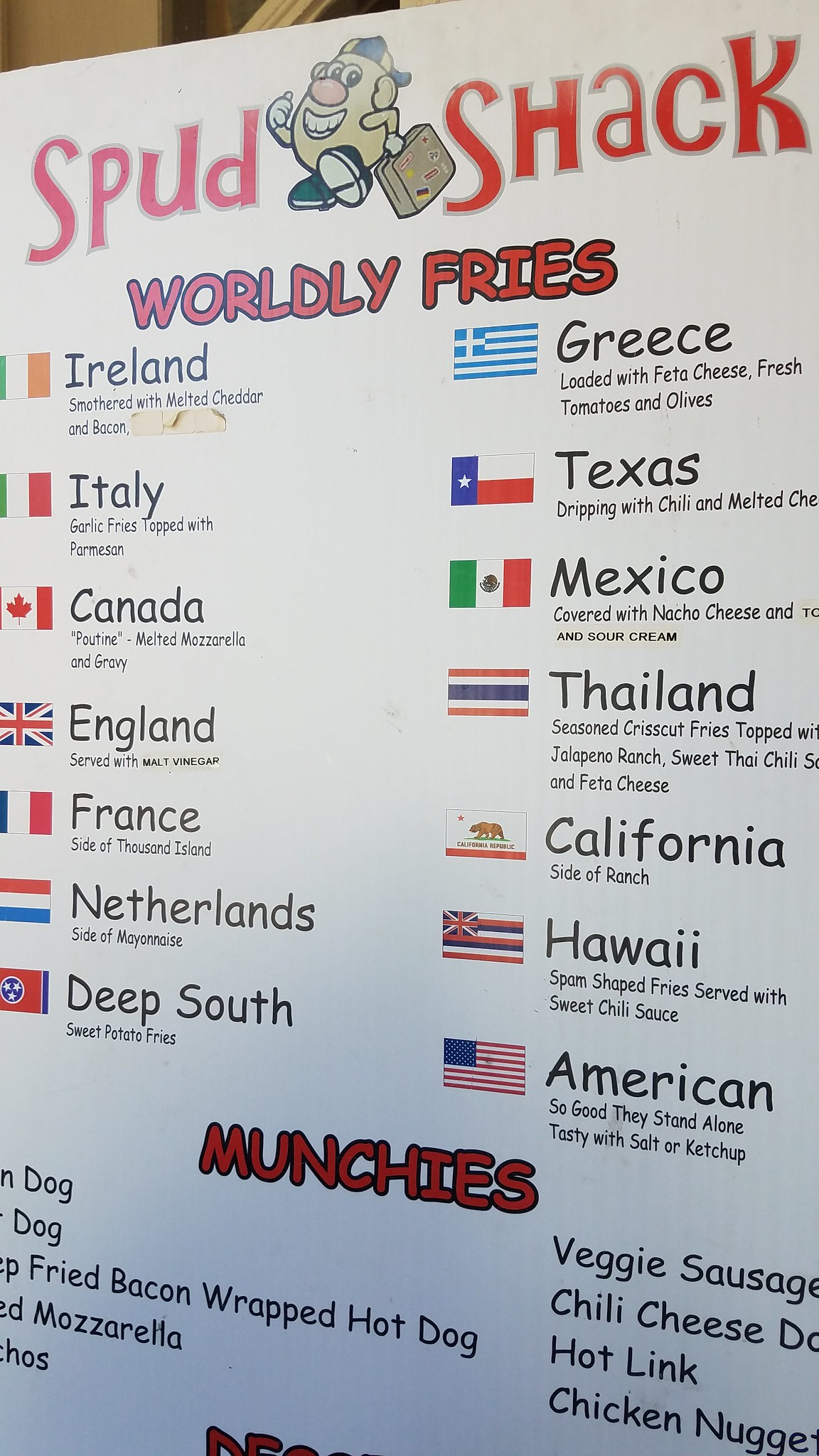**Spud Shack Menu**

Welcome to Spud Shack, the ultimate destination for potato lovers! Our vibrant menu, centered around our playful mascot – a goofy cartoon potato character sporting a white smile, pink nose, lively eyes, a baseball cap, black shoes, and carrying a suitcase – showcases our global and state-inspired fry dishes. 

### Worldly Fries

In bold red font, our "Worldly Fries" section highlights an enticing array of dishes, each paying homage to a different country's or state's culinary heritage. Accompanied by their respective flags and listed in black font, our selections include:

- **Ireland:** Classic fries topped with savory Irish cheddar and crispy bacon bits.
- **Italy:** Fries garnished with robust marinara sauce, mozzarella cheese, and sprinkled with Italian herbs.
- **Canada:** Our take on poutine – fries smothered in rich gravy and cheese curds.
- **England:** Crispy fries served with a tangy malt vinegar and sea salt seasoning.
- **France:** French-inspired fries drizzled with creamy béchamel sauce and grated Gruyère cheese.
- **Netherlands:** Delicious fries with satay sauce and chopped onions.
- **Deep South:** Southern-style fries topped with BBQ pulled pork and coleslaw.
- **Greece:** Loaded with crumbled feta cheese, fresh tomatoes, and kalamata olives.
- **Texas:** Hearty fries with beef chili, gooey melted cheese, and jalapeños.
- **Mexico:** Zesty fries adorned with spicy chili lime seasoning, avocado, and salsa.
- **Thailand:** Fries paired with a tangy sweet chili sauce.
- **California:** Fries served with smashed avocado and lime.
- **Hawaii:** Fries complemented by sweet chili sauce.
- **American:** Classic American-style fries with a side of ketchup.

### Munchies

Under another vibrant red heading, our "Munchies" section offers a variety of delectable side dishes. Indulgent and satisfying options include:

- **Chili Cheese Dogs:** Juicy hot dogs smothered in chili and melted cheese.
- **Hot Links:** Spicy hot links perfect for a bold flavor kick.
- **Chicken Nuggets:** Crispy chicken nuggets, golden-fried to perfection.
- And much more!

Dive into Spud Shack’s diverse menu and take your taste buds on a journey around the world with our unique and flavorful fry-centric dishes!